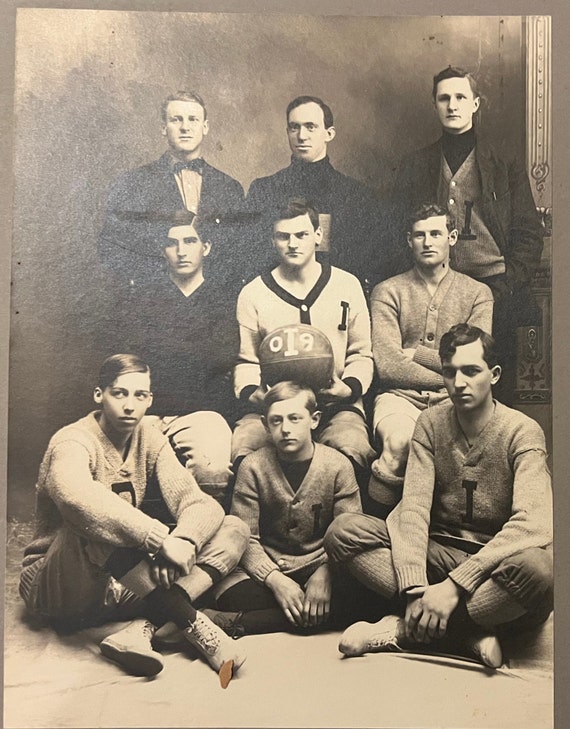This black-and-white, sepia-toned photograph captures a meticulously posed group, likely from the early 1900s, comprising nine males of varying ages, arranged in three rows. Standing in the back row are three men, presumed to be coaches or faculty, dressed in formal attire: suits and ties, with one sporting a bow tie and another a turtleneck paired with a suit jacket. Seated in the middle row, three young men occupy chairs, with the central figure holding an old-fashioned ball, possibly a rugby ball, marked with the letters "O," "9," and a prominent "I." This central individual, along with his two companions beside him, dons a sweater featuring an embroidered "I," suggesting affiliation with a school or university. Positioned in the front, three boys sit cross-legged on the floor, each wearing sweaters with the same "I" emblem, casual pants, and shoes. Their youth and attire indicate they are likely athletes or students. The diverse ages within the group, coupled with the formal wear of the men in the back, hint at an institutional setting, possibly a boarding school or a sports team photograph taken in a professional studio with a Victorian backdrop.